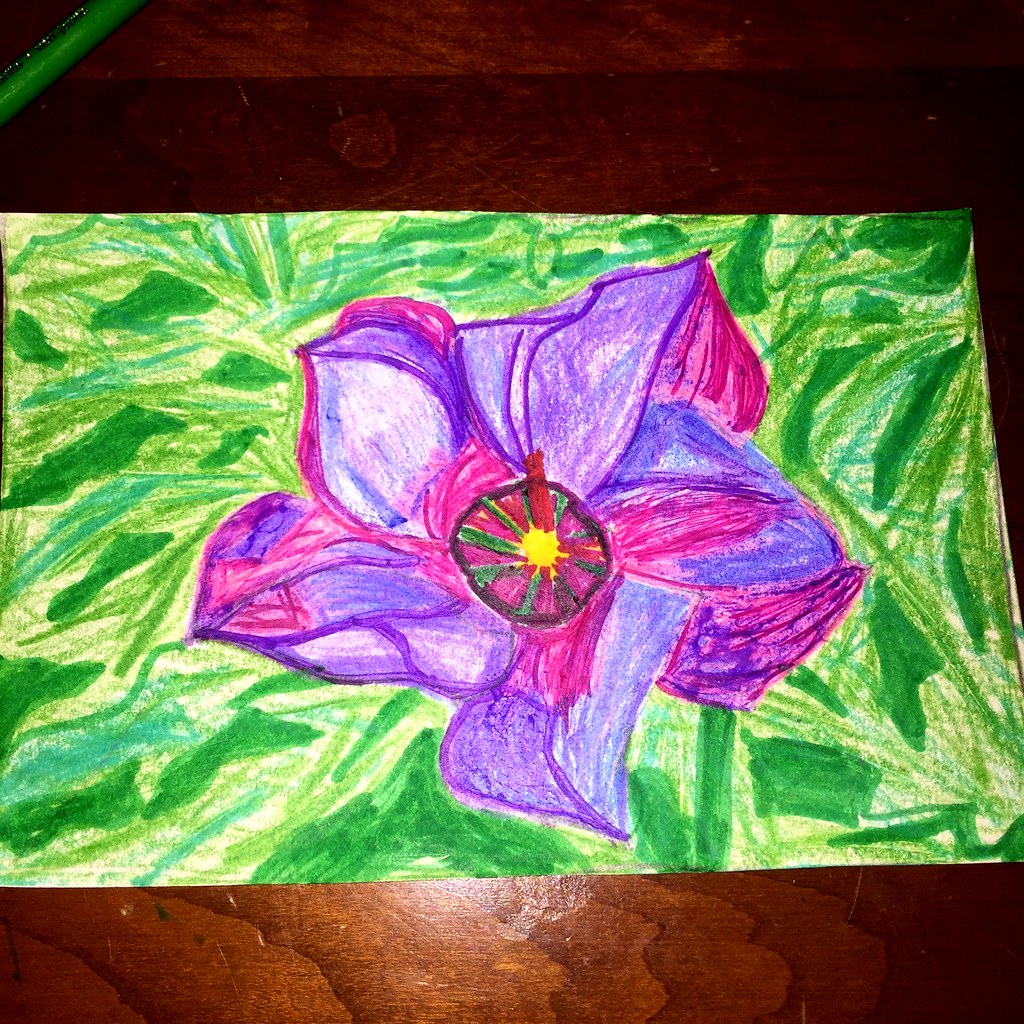A large, vividly colored drawing of a flower, created using markers and colored pencils, is captured in this color photograph. The flower, set against a backdrop of vines and various shades of green foliage, dominates the composition. The intricate design features a striking pink center with green stripes radiating outward like the spokes of a wagon wheel, converging into a yellow dot with a pink cylinder extending from it. Surrounding this center are five or six pointed petals shaded in hues of purple, blue, and pink. The artwork, occupying most of the photograph's height and nearly its entire width, appears to be placed on a dark wooden table, with a patch of light illuminating the surface at the bottom. The detailed foliage, rendered in at least three different shades of green, adds depth and frames the vibrant flower, giving the piece a lively, natural setting. The overall effect is one of youthful creativity combined with careful detail, ensuring the vivid flower stands out against its lush, green background.